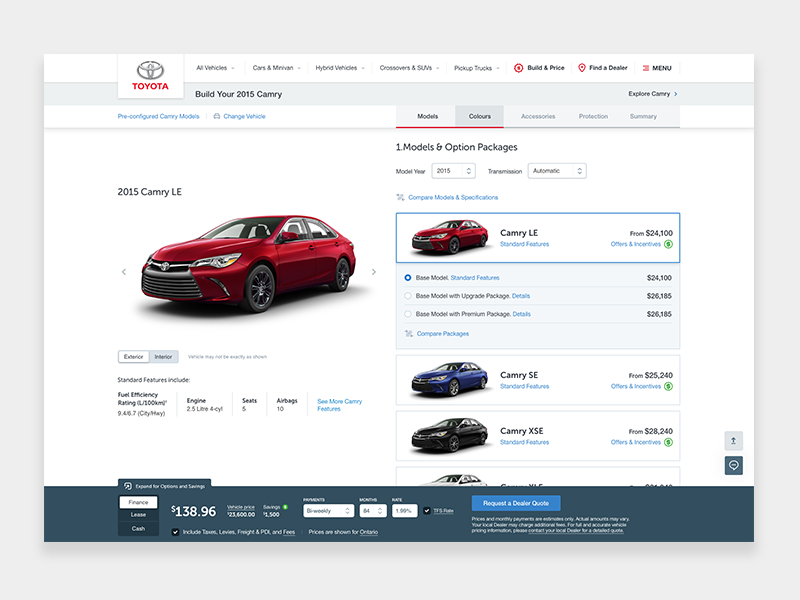Screenshot of the Toyota website showcasing the 2015 Camry LE. The upper left corner displays the Toyota logo followed by the word "TOYOTA" in bold red capital letters. The top navigation bar includes options: "All Vehicles," "Cars & Minivans," "Hybrid Vehicles," "Crossovers & SUVs," "Pickup Trucks," "Build & Price," "Find a Dealer," and "Menu."

Directly beneath the navigation bar, text reads "Build Your 2015 Camry," with additional options for "Pre-Configured Camry Models" and "Change Vehicle." Below this, the "2015 Camry LE" title is prominently displayed alongside an image of a red sedan. Standard features are listed as fuel efficiency rating, engine type, seating capacity of five, and ten airbags. A blue link invites users to "See More Camry Features."

On the far right, the page details "Models and Option Packages" with "Model Year: 2015" and "Transmission: Automatic" selected. A blue-framed box features another image of the car, specifying "Camry LE Standard Features from $24,100" along with "Offers and Incentives." The base model's standard features are listed at $24,100. Below this, images of additional models include a blue sedan labeled "Camry SE from $25,240" and a black sedan labeled "Camry XSE from $28,240."